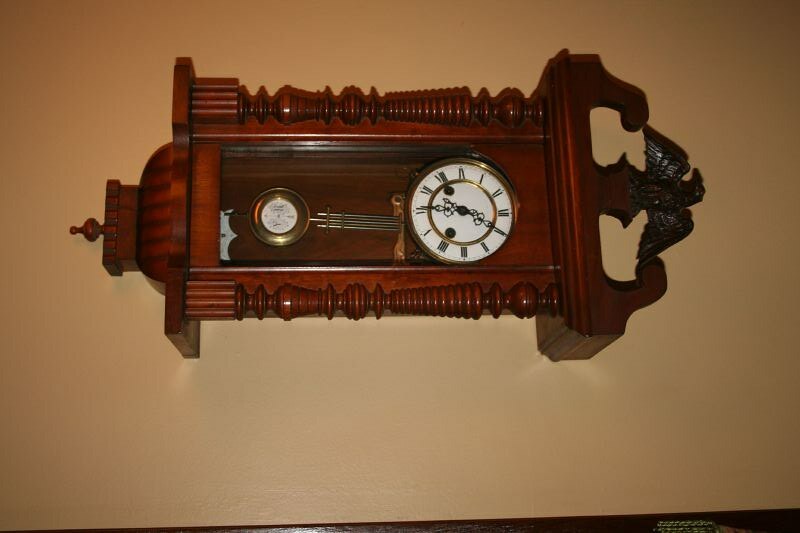A detailed photograph showcases an ornate wall clock mounted on a beige wall. The clock is large and rectangular, crafted from dark wood, and the photo appears to be taken with the camera sideways. The clock's intricate design features a carved bird perched at the top and decorative, pillar-like legs adorned with circular notches. The clock face is white, encircled by a gold ring, and displays black hands. There is no text present within the image.